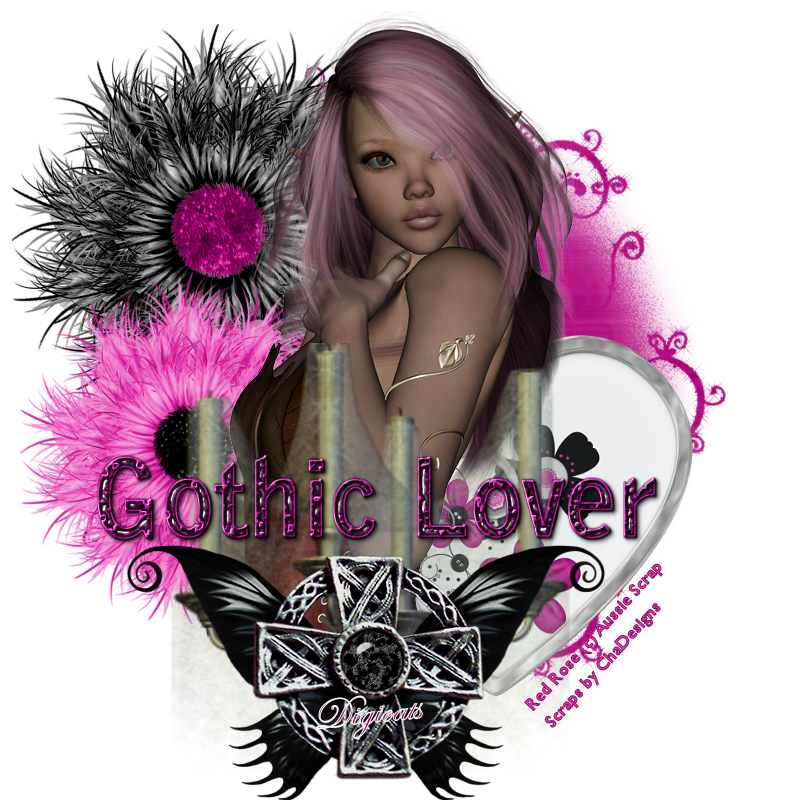The image displays a computer-generated African-American woman with shoulder-length, light pink hair, and hazel eyes looking slightly upward. She's depicted with a 3D texture, giving her skin a plasticky appearance. Her lips are puffy and light pink, forming a smooching gesture. Her attire is a brownish dress, covering the top half of her body, with intricate designs around the chest area, making it difficult to see beneath.

To the left of her, there are AI-generated black flowers with vivid pink centers and a swirling, circular design below them. To the right, a partially visible white or light gray valentine heart can be seen, accompanied by some purple scrollwork. At the bottom, a silver pendant with black and gray details forms a cross, adorned with black butterfly wings emerging from its sides.

The image includes several texts and logos: "Photo Bucket" is written in white font across the center, along with its circular logo. Below it, the words "Protect more of your memories" appear on a semi-transparent white banner. The phrase "Gothic Lover" is centrally placed in a pinkish-black shade. In the bottom right corner, there is a credit that reads "Red Rose Aussie Scrap Scraps by Cha Designs," adding a final touch to the composition.